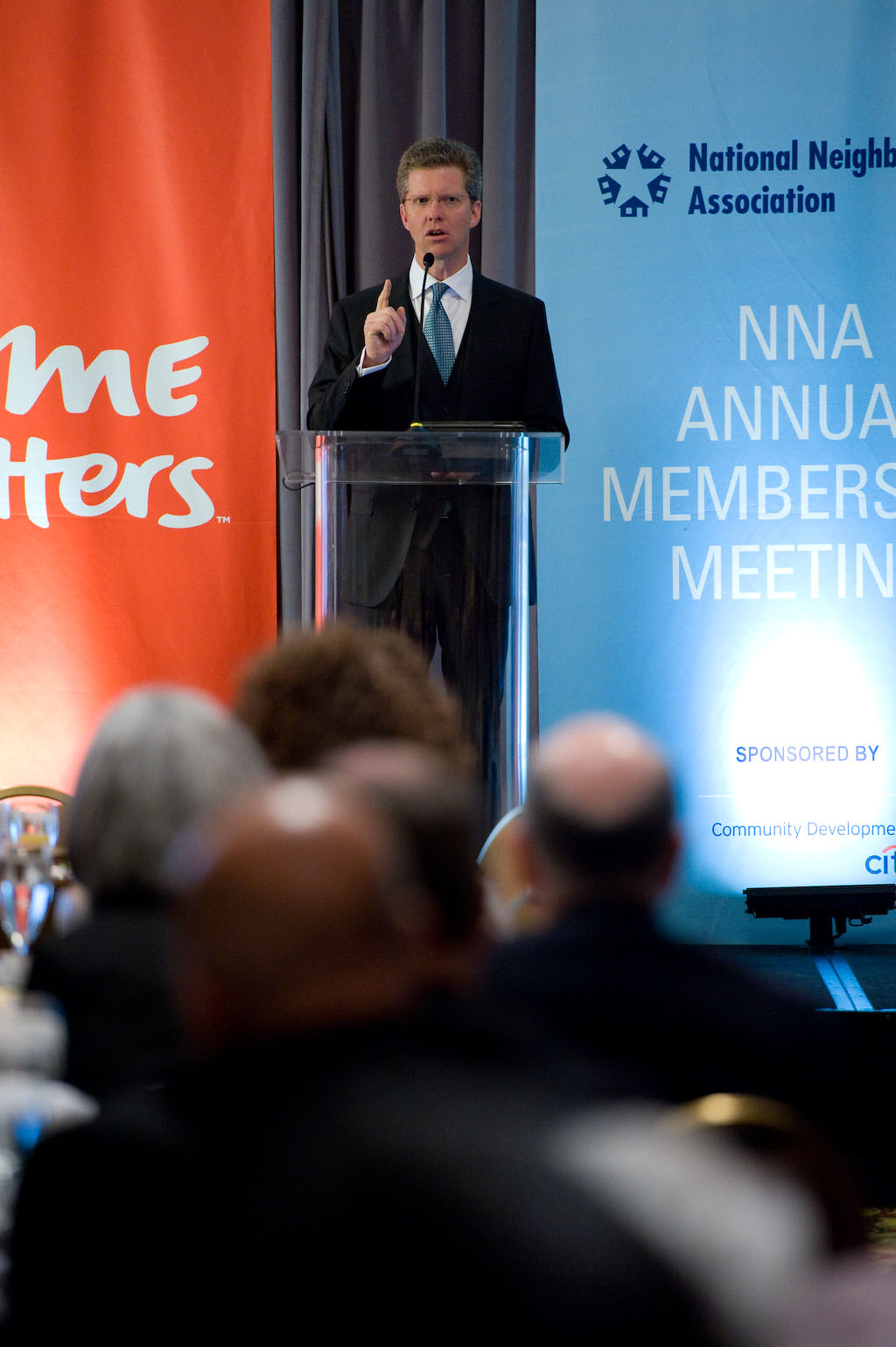In the image, a middle-aged Caucasian man is seen standing at a clear podium on a stage during a business conference, specifically the National Neighbors Association (NNA) Annual Membership Meeting. He is dressed in a black suit, white shirt, and blue tie, and is captured mid-speech with his hand raised, pointer finger extended, emphasizing a point. The backdrop features a black curtain and two distinctive banners. The banner to his right is blue and reads "National Neighbors Association NNA Annual Membership Meeting" with sponsor logos including Citibank. The banner to his left is reddish-orange, possibly indicating "Home Matters," though the text is partially obscured. The audience, slightly blurred and out of focus, consists of both men and women, with details like a woman with a gray bob and some balding men discernible. A stage light illuminates the speaker, drawing attention to his central role in the event.